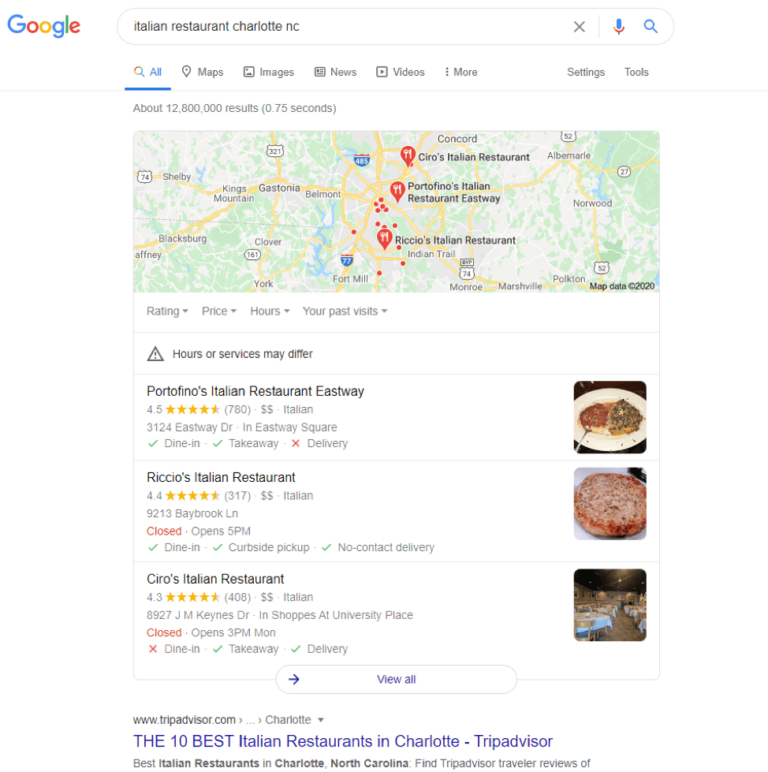The screenshot shows a Google search results page for the query "Italian restaurant Charlotte, North Carolina." The search bar at the top displays the entered query. Below it, there are three restaurant entries listed:

1. **Name**: Richio's Italian Restaurant (spelling unclear due to small text)
   **Location**: Eastway
   **Website**: www.tripadvisor.com

2. **Name**: Riccio's Italian Restaurant
   **Location**: Not specified
   **Website**: www.tripadvisor.com

3. **Name**: Ciro's Italian Restaurant
   **Location**: Not specified
   **Website**: www.tripadvisor.com

Each listing includes a small picture beside the restaurant's name. Above the list of restaurants, there is a caution sign, represented by a triangle with an exclamation mark, warning users that "hours of service may differ."

At the very top of the page, the menu options are displayed, with "All" currently selected, highlighted by a blue underline. Other options in the menu bar include Maps, Images, News, Videos, More, Settings, and Tools. Additionally, the website www.tripadvisor.com is referenced multiple times, indicating the source for "The 10 Best Italian Restaurants in Charlotte."